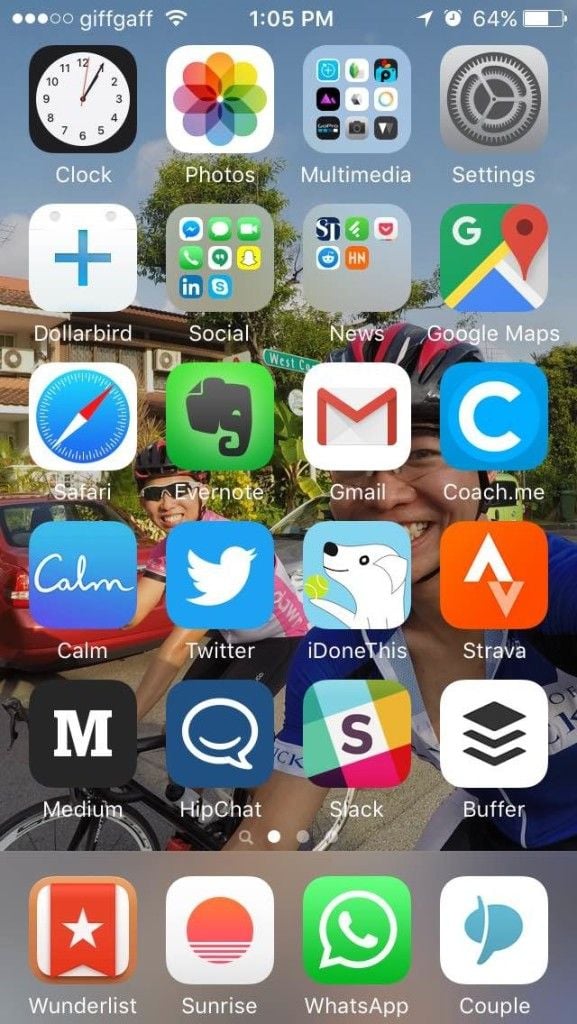A detailed screenshot of a smartphone home screen showcasing a vibrant and lively background featuring two individuals riding bicycles. Both riders are equipped with helmets and sunglasses, and they appear to be enjoying their time outdoors. Over this energetic backdrop, multiple application icons are neatly arranged:

1. At the top, there's a rectangular widget displaying a clock icon, labeled "Clock."
2. Next, we see a white square icon with a blue cross, labeled "Dollarbird."
3. A blue square icon featuring a prominent white "C" is labeled "Coach.me."
4. Another blue square icon simply says "Calm" in white text with the same label beneath it.
5. A blue square with a white bird icon is identified as "Twitter."
6. Following this, there's a light blue square with an image of a white dog, whose face is partially visible, highlighting one black eye, nose, smile, ear, and a raised paw holding a tennis ball. This is labeled "iDoneThis."
7. A black square icon featuring a large white "M" is labeled "Medium."
8. Finally, a green square with a white text bubble and a phone icon is labeled "WhatsApp."

The neatly arranged array of app icons over the dynamic biking background creates a lively and functional home screen.